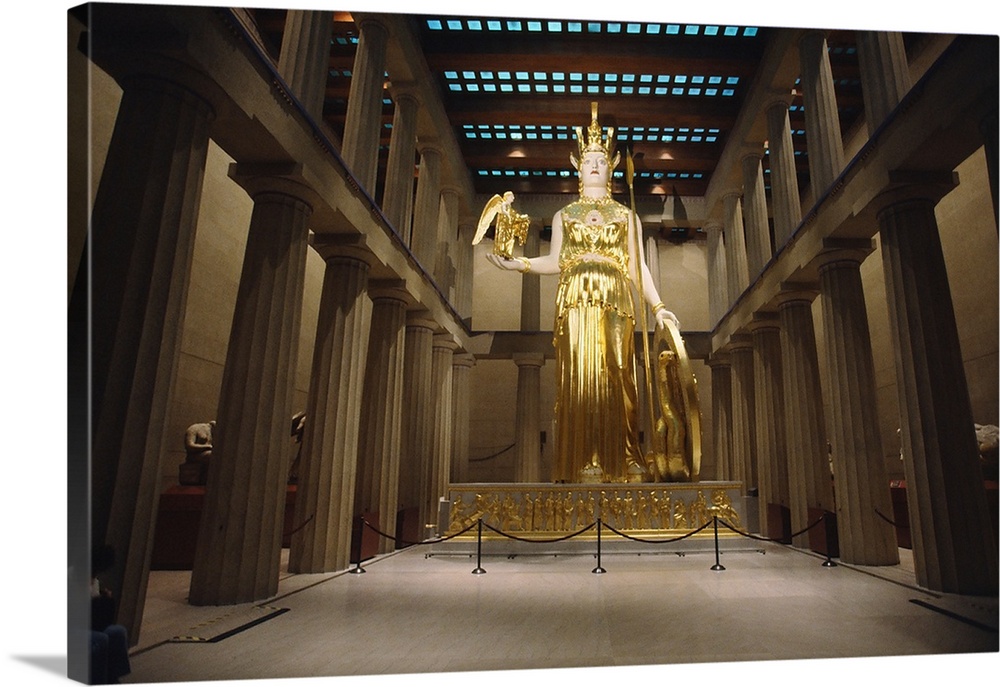The color photograph captures the interior of what appears to be a carefully curated museum exhibit, designed to emulate an ancient temple or church. Dominating the center of the composition is an imposing statue of what seems to be a goddess or deity. This elaborate sculpture portrays a tall woman with pale skin, adorned in a resplendent, solid gold dress that leaves her shoulders exposed but covers the rest of her form down to her feet. She is crowned with a helmet and stands on a large, rectangular white base decorated with intricate golden figures.

In her right hand, she holds a golden angel or eagle with its wings outstretched, palm up, adding to her commanding presence. Her left hand grasps a large wheel-like object, angled slightly, with a serpent seemingly interwoven between her and the wheel, as though hugging against it. Resting against her shield-bearing arm is a long spear, almost reaching the top of her head, further emphasizing her grandeur.

The statue is surrounded by a double row of classical marble columns, creating an imposing frame for the scene. The floor appears to be white marble, enhancing the opulent atmosphere. These columns rise to support a flat platform that encircles the room, beyond which stand additional smaller statues on red plinths, hinting at the room’s extensive collection. The entire scene is bathed in light from above, illuminating the golden statue and making it shimmer against its detailed backdrop, all while being set apart by a velvet rope that underscores its significance within the exhibit.